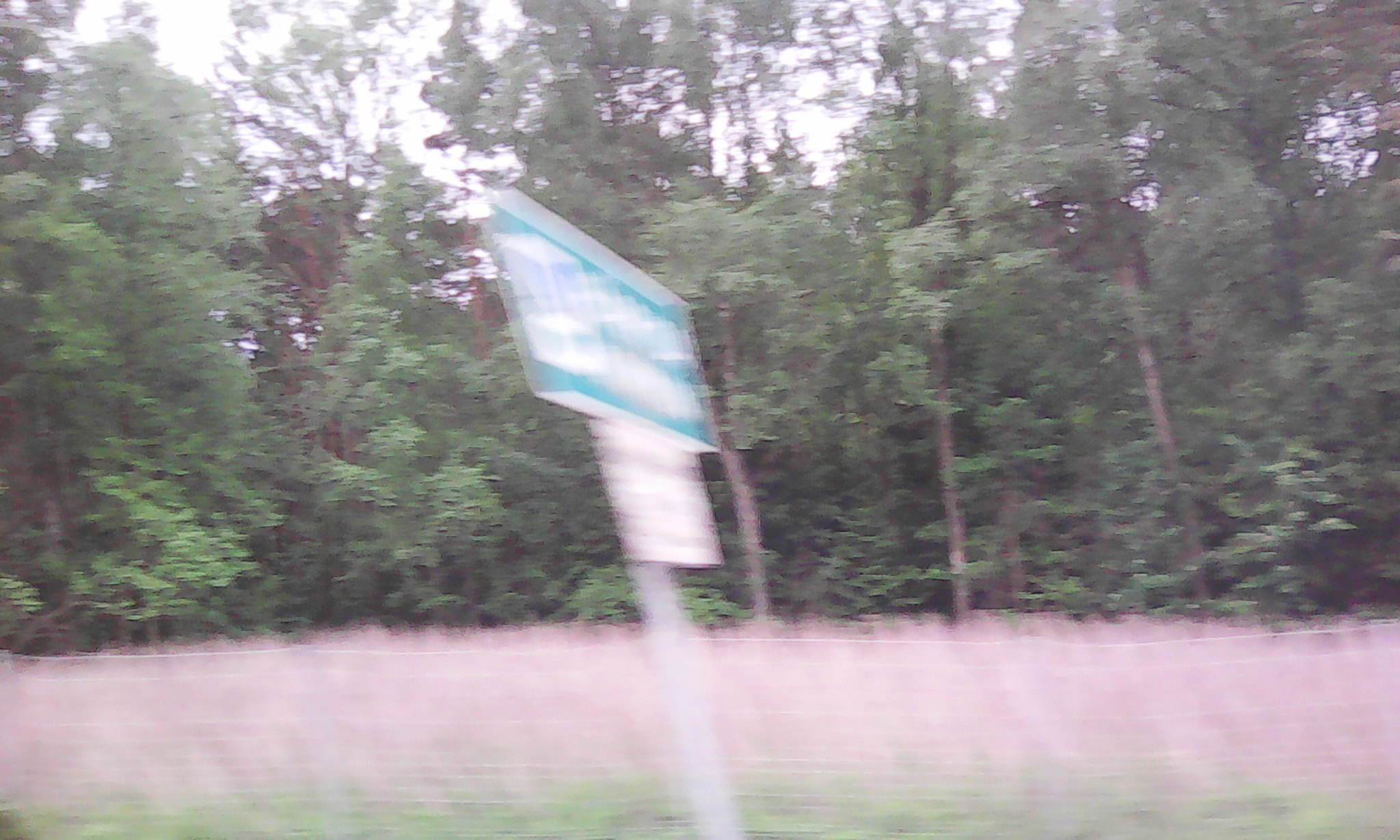The image captures a blurry scene, seemingly taken from a moving vehicle, depicting a slightly tilted green and white road sign. The larger, green sign with illegible white text sits above a smaller white sign, both mounted on a metal pole. Behind the signs, a fence stands in front of a patch of whitish-brown grass, transitioning into a section of green grass. The background consists of a dense, forested area under a bright, overexposed sky.